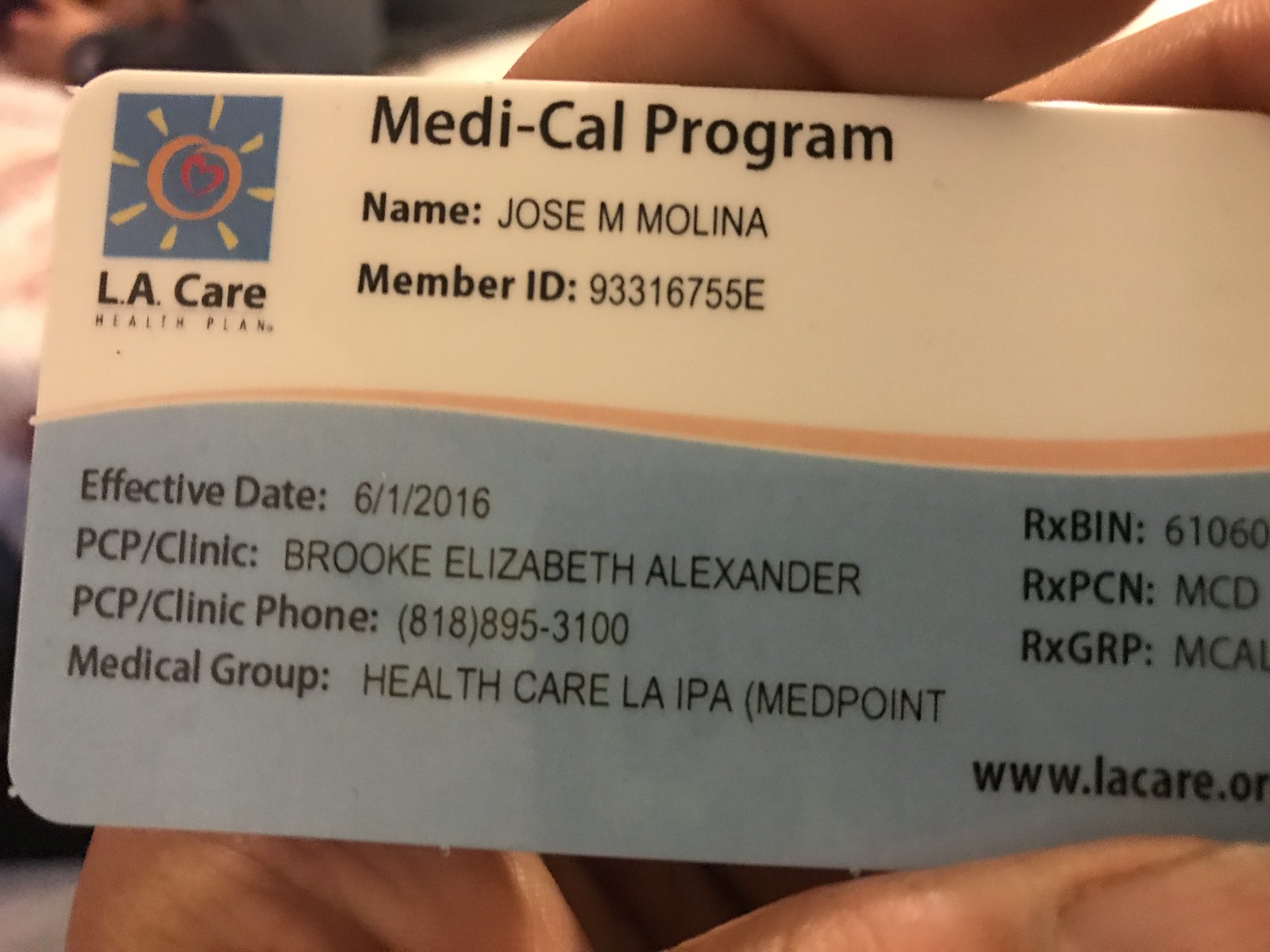This detailed color photograph captures a close-up view of an insurance card held in someone's hand. The card is associated with the LA Care Health Plan's Medi-Cal program. Featured prominently at the top left is the program's name. Below that, the card identifies the member as Jose M. Molina, with a member ID of 93316755E. The card indicates an effective date of June 1, 2016. The primary care provider (PCP) clinic listed is Brooke Elizabeth Alexander, and the clinic’s contact number is 818-895-3100. Additionally, the card mentions that the associated medical group is Health Care LA IPA MedPoint.